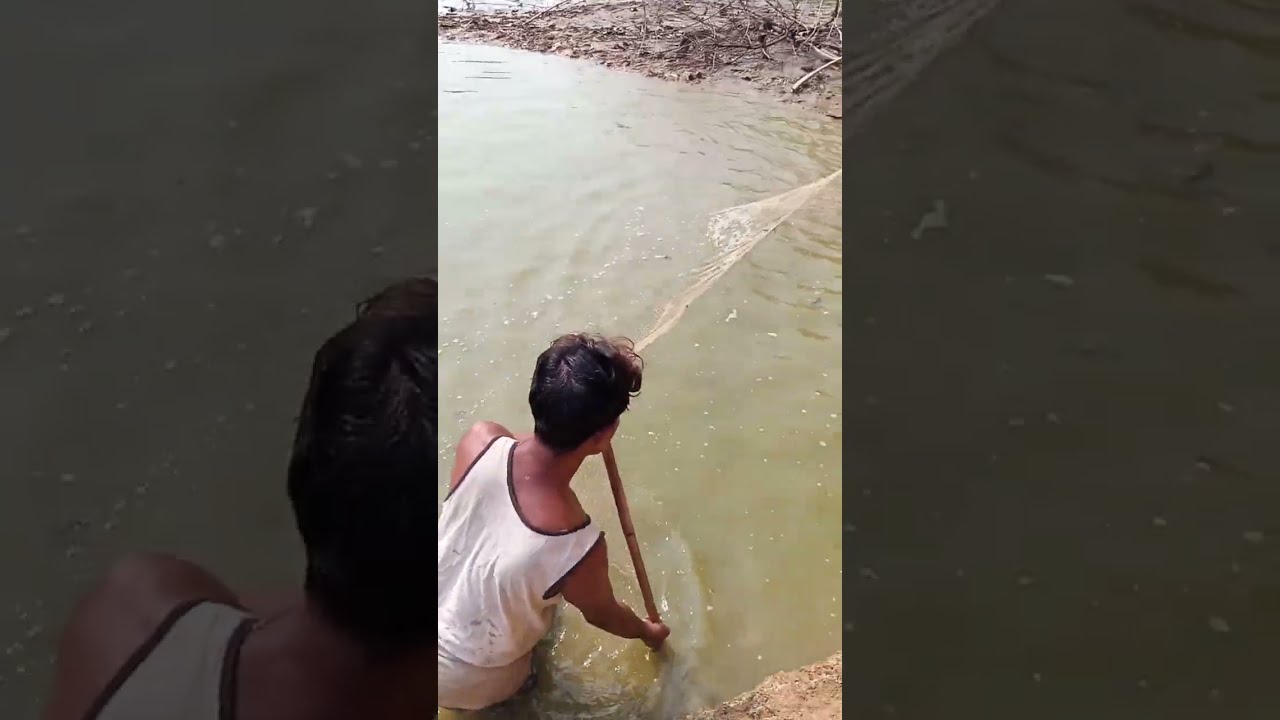The photograph captures an outdoor scene featuring a young boy, possibly a teenager, positioned from an above-and-back angle while standing or crouching in knee-deep, murky, brownish-green water that appears almost muddy. His short, very dark hair and a white sleeveless tank top with black stitching are prominent, and he is seen handling a thick, smooth bamboo or wooden pole, akin to a large straw. This pole, possibly part of a fishing net or similar apparatus, extends into the water as if he is attempting to catch something, likely fish. The surroundings in the image include a muddy, dark brown coast with scattered, dead branches, enhancing the sense of a natural but untidy environment. His lower attire seems to be tan-colored shorts or pants, partially submerged in the muddy water, adding to the scene's overall earthy and gritty ambiance.